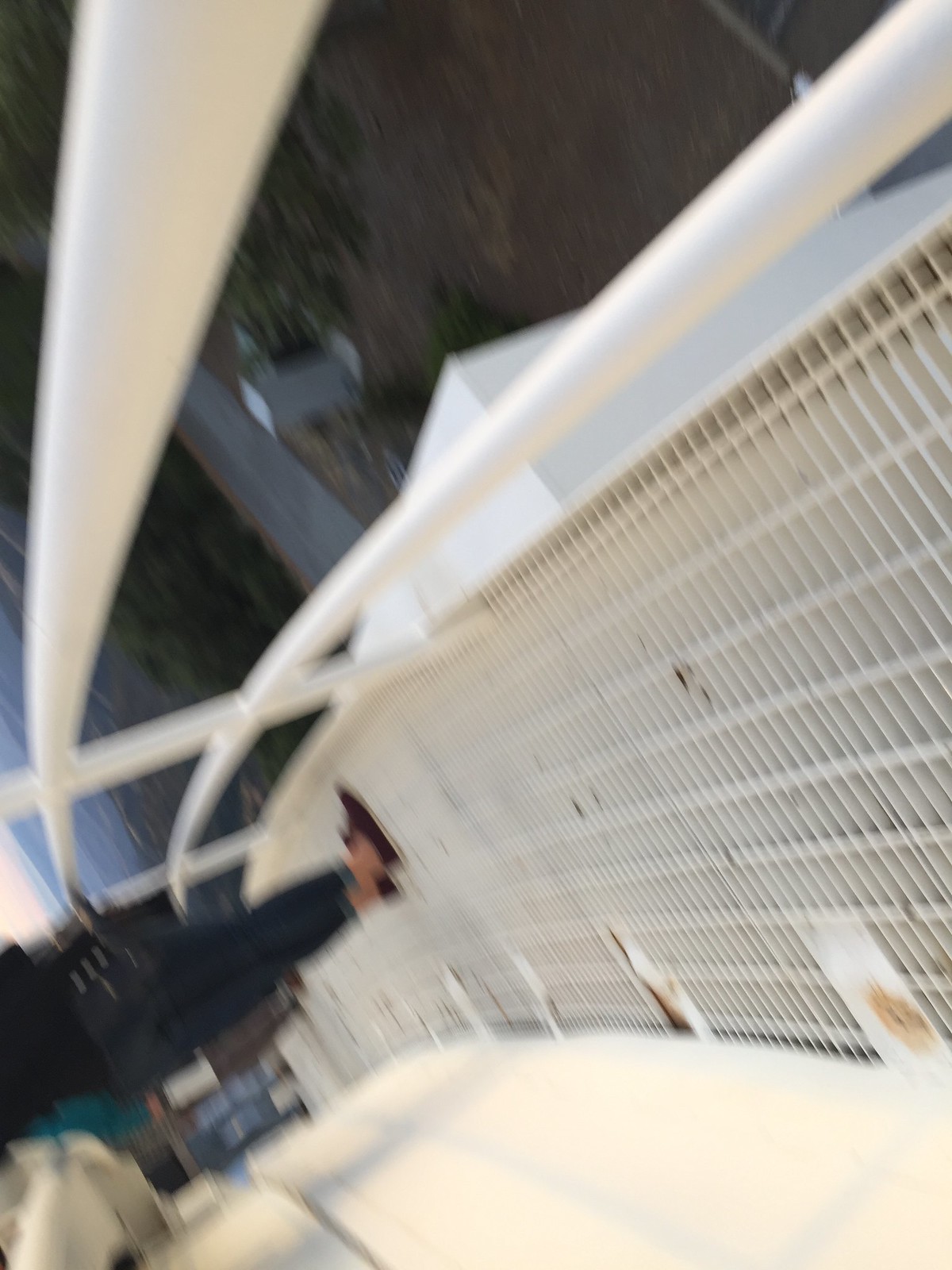A blurry photograph of an outdoor scene, rotated 90 degrees anti-clockwise, showing a person standing on a white metal ledge. The image captures the individual from the torso down, partially obscuring their identity. The ledge features white railings, through which the distant ground is visible, emphasizing the height of the platform. The grated surface of the ledge allows a partial view to the area below. In the background, trees and a road can be faintly discerned, adding context to the elevated position of the scene.